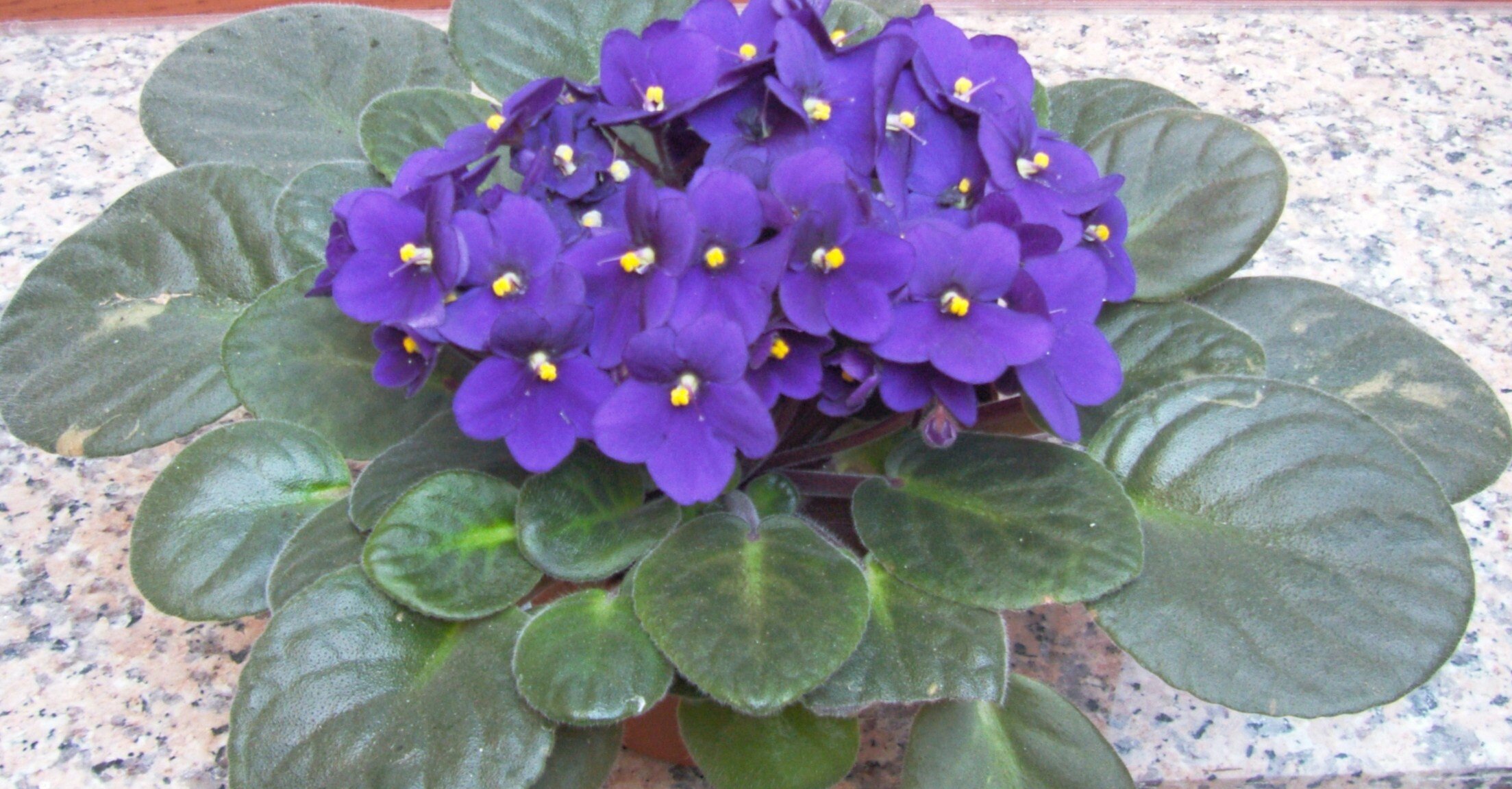The image showcases a vibrant and large African Violet plant thriving in a ceramic pot on a visually striking marble countertop. The lush plant boasts an array of deep blue-purple, or "blurple," flowers, numbering around thirty, each adorned with a tiny yellow center. Surrounding these flowers are numerous green leaves of varying sizes, some glossy and new, while others appear slightly dusty. The leaves exhibit a rich, dark green hue with patches of brighter green and occasional white discolorations, and their shapes are mostly rounded and somewhat oval. The marble countertop beneath is predominantly white with intricate flecks of blue, pink, gray, and orange, adding a sophisticated depth to the scene. In the background, just a sliver of the terracotta-colored wall can be seen, hinting at a warm ambiance without detracting from the plant's commanding presence. Overall, the African Violet plant occupies the majority of the frame, creating a lush and captivating focal point.